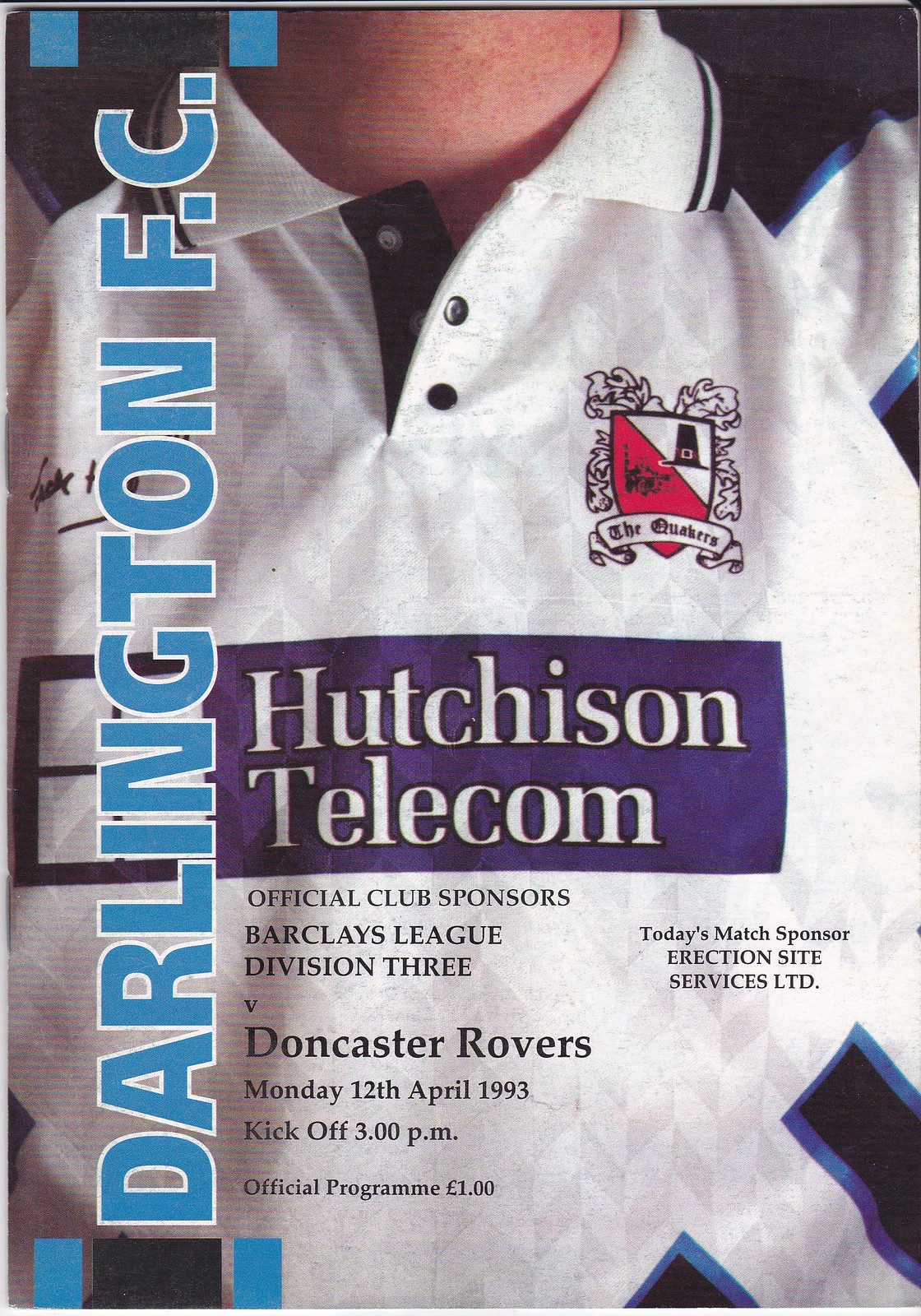The image features a magazine cover showing a person from the neck down to their torso, emphasizing their white polo shirt with black and blue trim. Prominently displayed on the shirt is a logo: a white and red shield with a pilgrim hat, white leaves, and a ribbon that reads "The Quakers." Central to the cover in a blue bar is the text "Hutchinson Telecom," denoting the official club sponsor of Barclays League Division Three. To the side, large letters spell out "Darlington FC" vertically in blue. Further details announce a match against Doncaster Rovers on Monday, April 12th, 1993, with kickoff at 3 p.m. This is identified as the official program for the game, priced at three pounds. Additionally, it mentions today's match sponsor as Erection Site Services LTD.